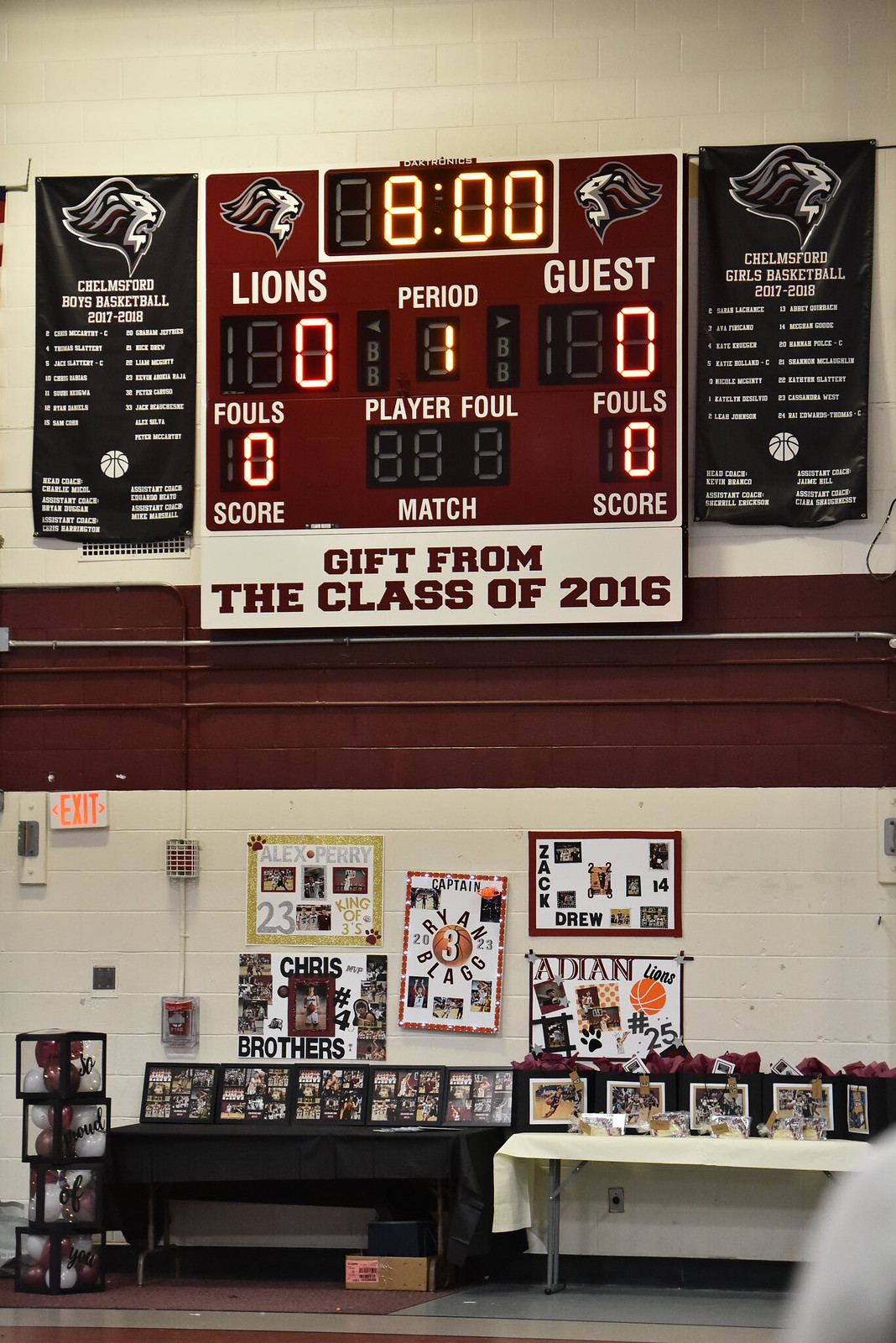The photograph captures the interior of a gymnasium, prominently featuring a square-shaped scoreboard that reads "Gift from the Class of 2016" at the bottom. The scoreboard, set against a maroon background, shows an 8-minute timer with both the "Lions" and "Guest" teams at 0, indicating it's the first period with no fouls recorded. Flanking the scoreboard are two banners depicting a lion's head, representing the Chelmsford boys' and girls' basketball teams, respectively. Beneath the scoreboard, the gymnasium wall displays numerous student-made banners and posters. In the foreground, there are two long tables covered in black and beige tablecloths, laden with various images and pictures, possibly for sale, set against a beige wall.